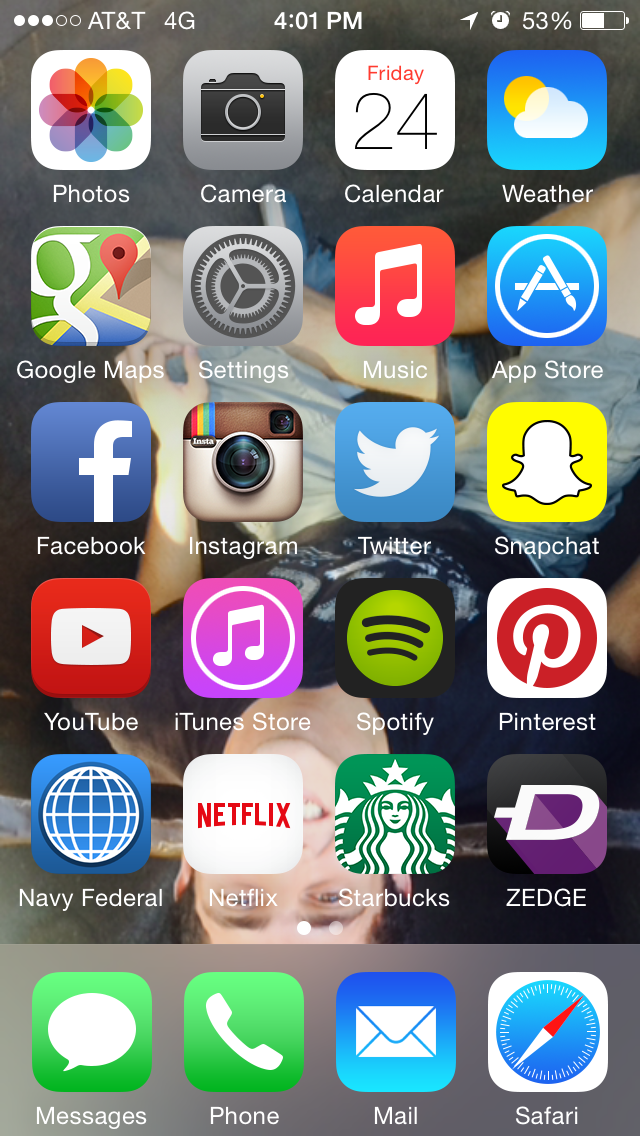The screenshot captures a mobile device’s home screen, showcasing a variety of apps arranged in a grid format. In the top-left corner, there is an AT&T 4G network signal indicator with three out of five circles filled. At the center of the top bar, the time is displayed as 4:01 PM. In the top-right corner, several icons are visible: a right-pointing arrow, a small alarm clock symbol, and a battery icon showing 53% charge, half-filled in white and half clear.

Directly below this status bar, the screen is arranged in rows of app icons. The first row features the Photos, Camera, Calendar, and Weather apps. The second row includes Google Maps, Settings, Music, App Store, and Facebook. The next row contains Instagram, Twitter, Snapchat, and YouTube. Further down, there are the iTunes Store, Spotify, Pinterest, Navy Federal, Netflix, Starbucks, and Zedge icons.

At the very bottom of the screen, four essential app icons are docked: Messages, Phone, Mail, and Safari, each represented by its respective iconic symbol.

The background of the screen is a personal photograph. The image is upside down, with a person’s head positioned near the bottom of the screen and their crossed legs near the top. The individual is smiling and looking up, dressed in a black shirt and gray shorts.